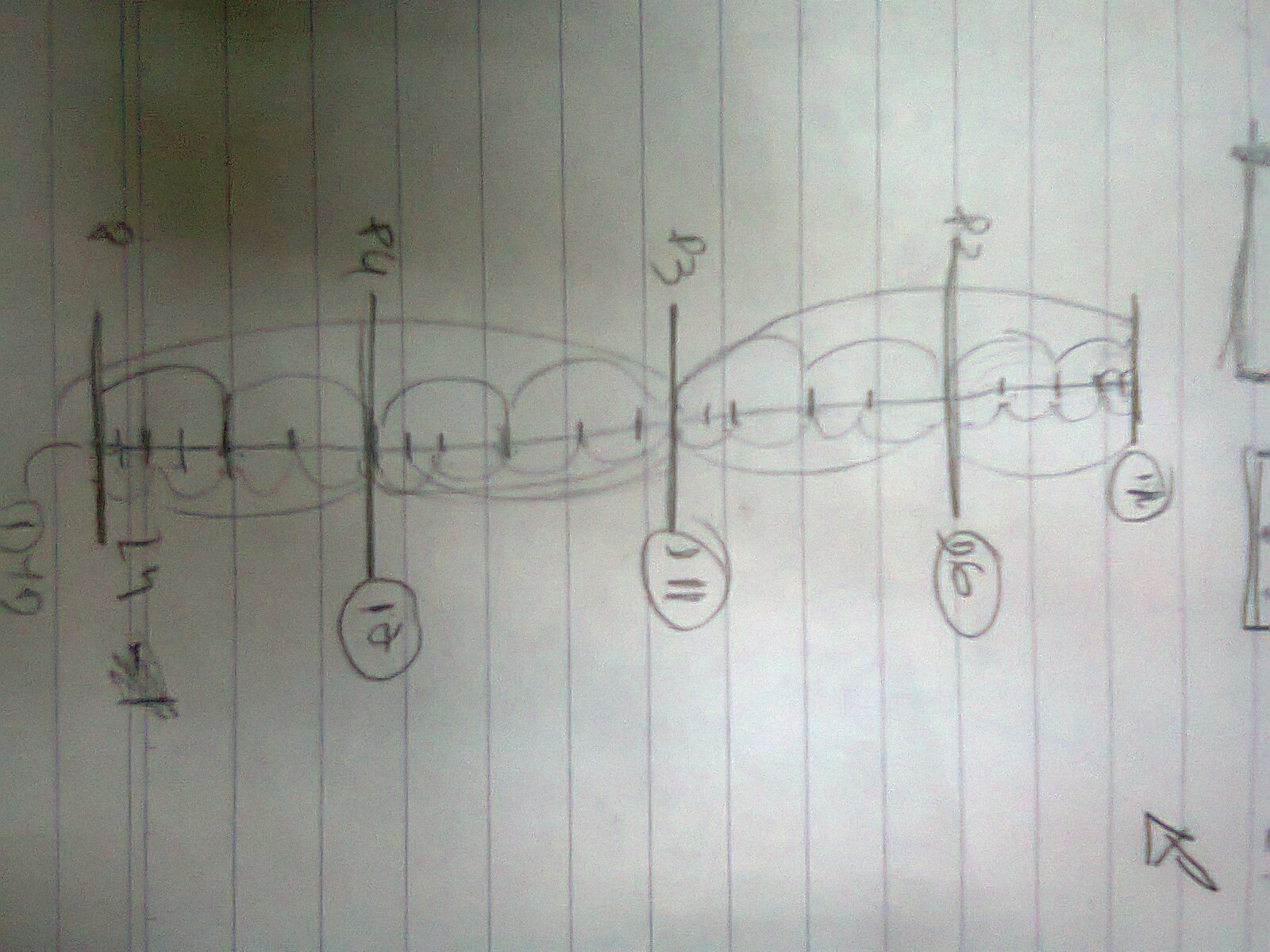The image, positioned horizontally on a lined piece of paper that was originally meant to be vertical, features a pencil drawing with darker shadowing towards the bottom. At the top of the page, there are two half squares that appear to be cut off. An arrow drawn in pencil points from the top right corner towards the middle of the page. The paper has five evenly distributed horizontal lines covering approximately the middle third of the page. At the very bottom, there are some hard-to-read numbers written on each side. The left number sequence from bottom to top is P4, P3, and P2, while the corresponding right side sequence is 12, 11, and 6. There is no P number on the very top line.